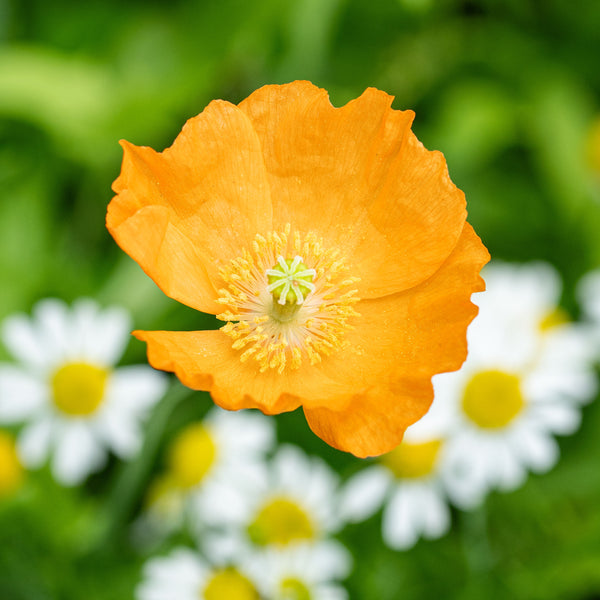In the foreground of this vibrant image is a spectacularly yellow flower adorned with striking burnt orange edges on its large petals. Emerging from the flower's vibrant center are numerous yellow and white buds, accompanied by a prominent green stem that further branches into smaller white buds. This contrasting palette of warm hues beautifully highlights the flower's intricate details. In the background, an out-of-focus garden scene frames the central flower, dotted with multiple white daisies, each featuring classic yellow centers. The greenery surrounding the daisies adds depth, creating a lush, springtime garden ambiance. The overall composition captures the essence of natural beauty with a detailed focus on the flower's structure and an inviting hint of its garden setting.